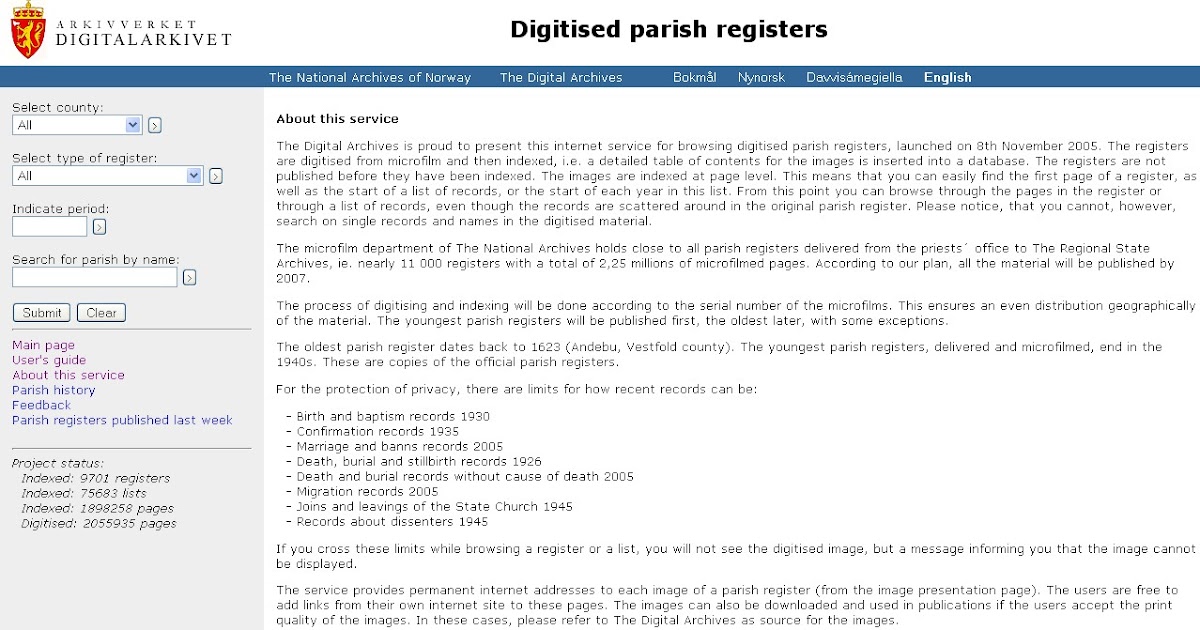**Detailed Descriptive Caption:**

This image illustrates an informative article about a digital service for accessing parish registers, presented by the Digital Archives. The article, written in black text on a white background, is centered on showcasing their digitization initiative. At the top of the page is the title "Digitized Parish Registers," indicating the subject of the article. 

To the top left, a red icon with a yellow diagonal line accompanies the text "Archivate – Digital Archivate." This branding highlights the digital nature of the service.

The description within the article elaborates on the Digital Archives' pride in launching this internet service for browsing digitized parish registers on November 8, 2005. These registers have been meticulously digitized from microfilm and indexed in a detailed table of contents inserted into a database, with indexing occurring at the page level. Thus, users can easily locate the first page of a register or the beginning of a specific list of records or yearly entries. However, the service does not permit searching for individual records or names within the digitized material.

Additionally, the article provides information about the extensive holdings of the National Archives’ microfilm department, which encompasses nearly 11,000 parish registers totaling 2.25 million microfilmed pages. A plan ensures that all material will be published by 2007, with a strategic approach to processing by microfilm serial number to maintain geographic distribution.

Historic details are shared, noting the oldest parish register from Andebu, Vestfold County dating back to 1623 and the youngest from the 1940s. Privacy protection measures are mentioned, stating that users cannot view digitized images if they contain recent records beyond specified limits.

The text also highlights that each image from a parish register has a permanent internet address, allowing users to create links from their own websites. These images can be used in publications if the quality is acceptable, with appropriate credit to the Digital Archives as the source.

On the left side of the image, a digitized menu written in blue and purple provides various options such as "Select country," "Select type of register," "Indicate period," "Search for parish by name," "Submit," "Clear," "Main page," "User's guide," "About this service," "Parish history," "Feedback," and "Parish register published this week."

Overall, the image captures a comprehensive overview of the digital service for accessing parish registers, facilitating research and historical studies while maintaining privacy and accessibility standards.